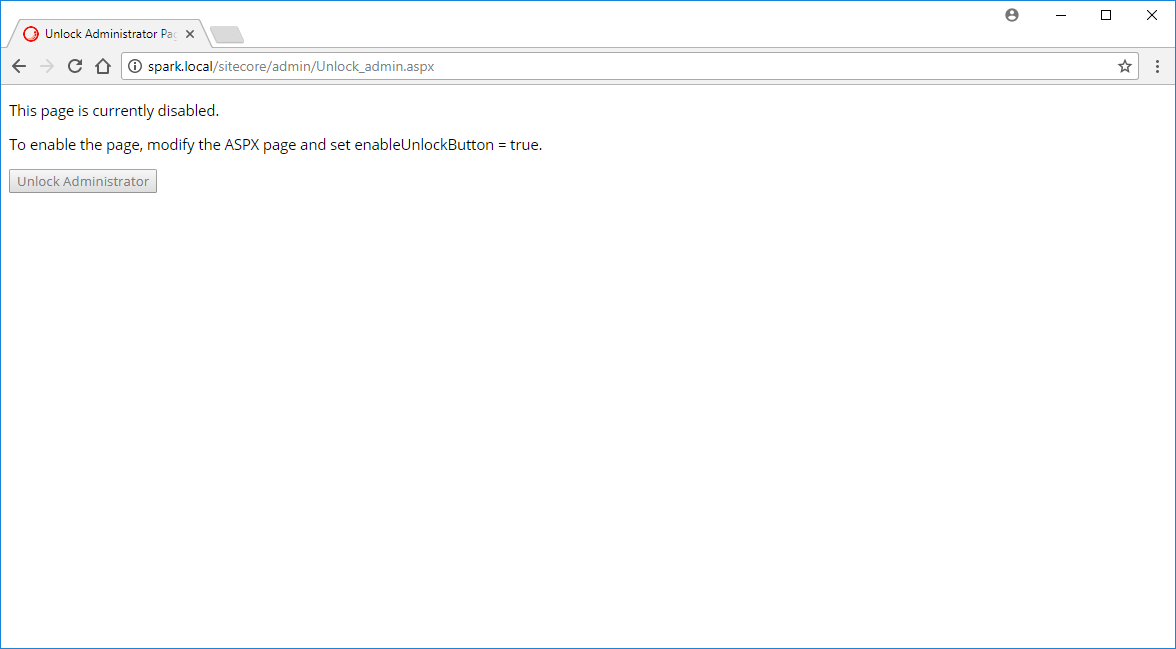The image depicts a user interface with various elements. On the right corner, there is a large white box outlined in blue. Inside this box, there is a small circle depicting a person, accompanied by a line, a square, and an 'X'. On the left side of the image, there is a blue tab featuring a red circle with white inside. Adjacent to this tab, the text "Unlock Administrator" appears next to an 'X'. Below this segment, there are left and right arrows, a circular arrow, an up arrow, and a search box. The contents of the search box read "spark.dot.local/sitecore/admin/unlockadmin.aspx" followed by a star and three dots. The white background contains the message: "This page is currently disabled. To enable the page, modify the ASPX page and set 'enableUnlockButton' equal to 'true'." At the bottom of the interface, there is a blue button labeled "Unlock Administrator."